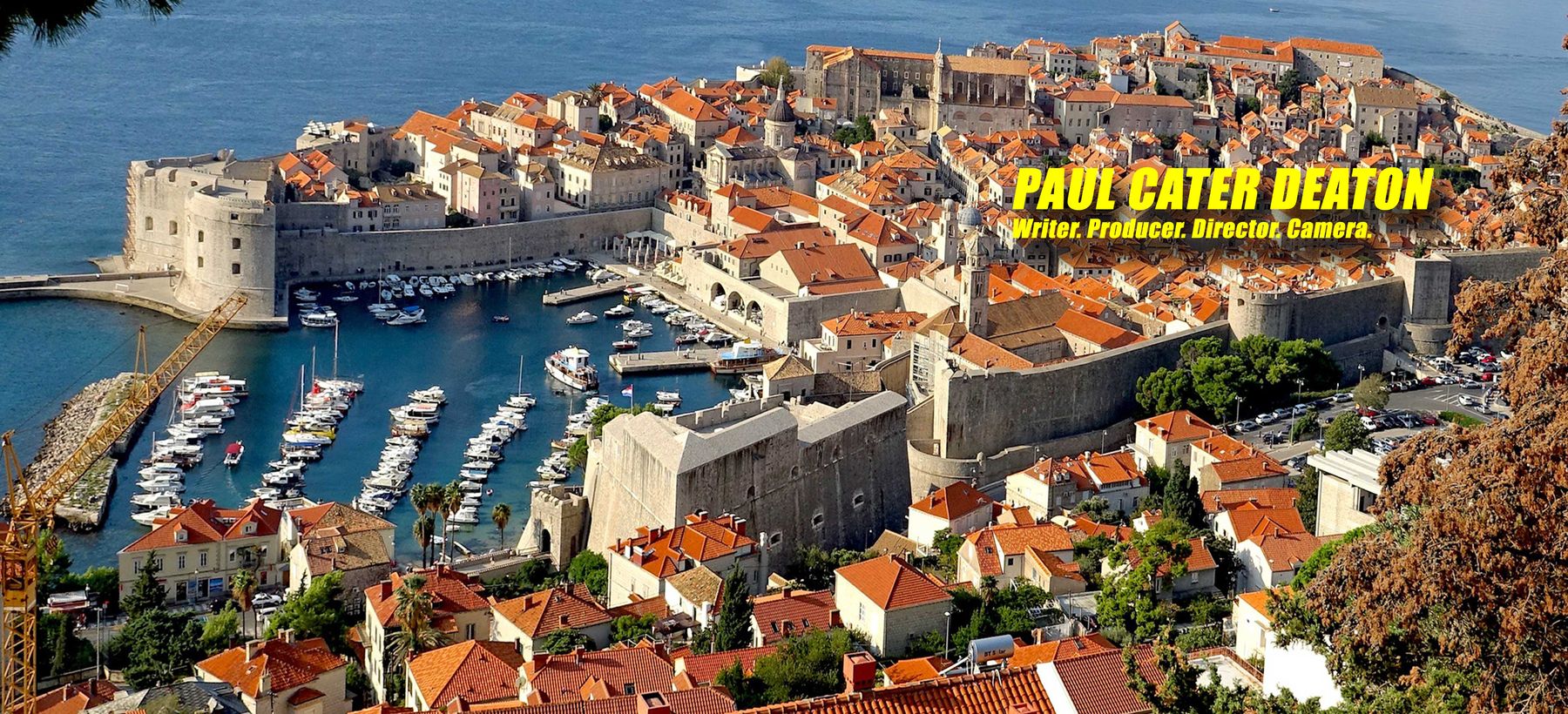The image is a narrow horizontal rectangle, showcasing an aerial view of the historic town of Dubrovnik, Croatia, which sits on the azure coastline. The town is densely packed with white stucco buildings topped with iconic red tile roofs. These structures are clustered closely together, forming a picturesque seaport village. Towards the left of the image, there's a bustling marina with numerous small boats docked and anchored, as well as several piers extending outward. The blue waters of the Adriatic Sea surround the town, enhancing its charm and offering a vivid contrast to the red roofs. In the top right corner of the image, there is gold text with a black shadow that reads "Paul Cater Deaton," with smaller text beneath it listing "writer, producer, director, camera." This image appears to be an advertisement for Paul Cater Deaton, showcasing his skills as he seeks employment. The photographic style is a blend of representationalism and realism, with the text giving it a professional and artistic touch.